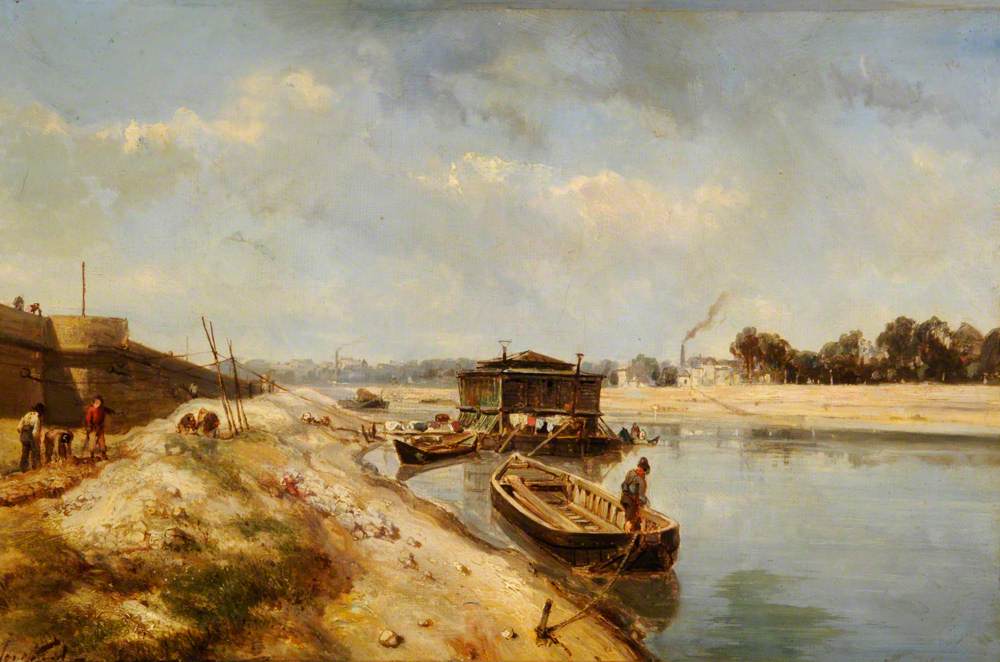The painting depicts a serene yet subtly bustling riverside scene. The sky is adorned with a blanket of clouds, with hints of smoke rising in the distance, possibly from factories, suggesting the early days of the industrial revolution. In the foreground on the right, a lone man sits in a small boat anchored by a wooden stake, holding onto the rope. The boat faces away from the viewer. Further into the river, there's a medium-sized boat and a large boat, the latter appearing industrial with smoke stacks indicating its steamboat nature.

The riverbank is dotted with green grass, sand, stones, and rocks. To the left on the shore, three individuals are visible—one bent over, while the other two stand nearby. Behind them looms a large boundary wall, perhaps fortifying a town. This townscape includes elevated land with two figures standing, observing the river. Beyond the immediate shore, more boats are visible, adding to the sense of activity on the river.

A square building with a small canopy sits on the water, adding architectural interest. In the far distance, trees and buildings, possibly factories with smoke billowing, line the opposite shore, merging with a hilly landscape, completing the industrious yet picturesque tableau.